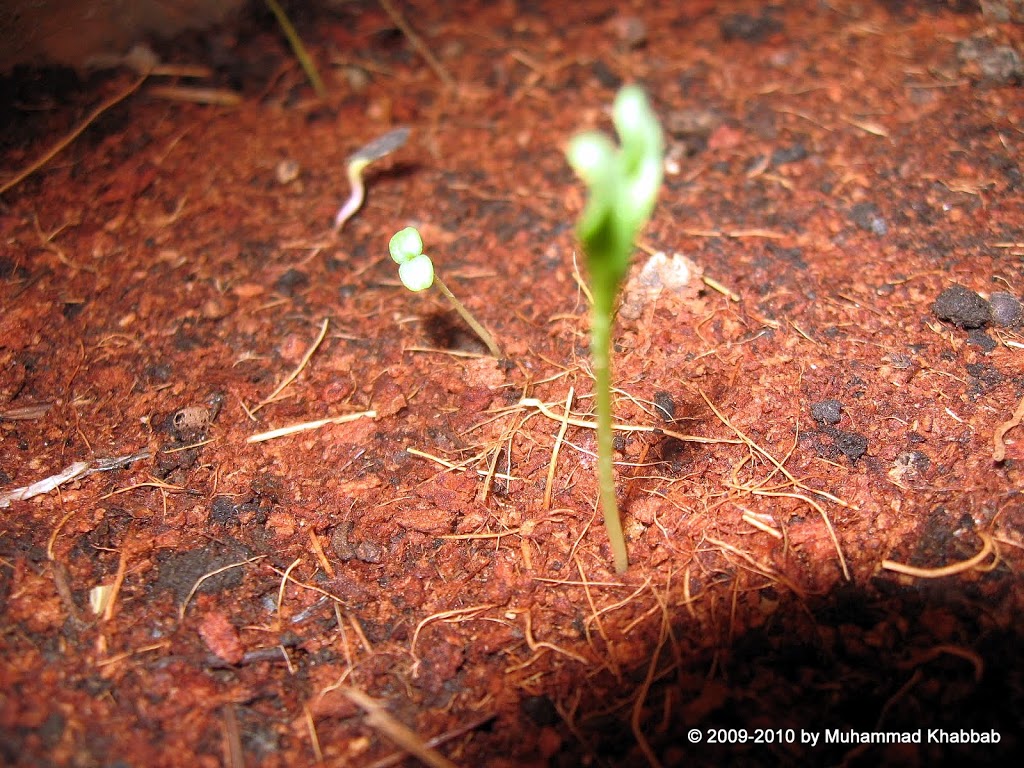This rectangular photograph, likely taken either indoors or at night due to its dark ambiance, prominently features a few freshly sprouted green seedlings growing from a mixed surface of red mulch and soil. The center of the image is illuminated by artificial light, casting a contrast between the bright green of the plants and the darker background. The most prominent seedling stands tall in the center, surrounded by smaller sproutings to its left. The bottom right-hand corner of the photograph is marked by a dark area containing white text, a copyright watermark that reads "© 2009-2010 by Mohamed Khabab." The overall setting suggests a close-up view of a garden bed, capturing the early stages of plant growth. The image composition includes scattered rocks and sticks, with the predominant colors being green, red, white, and shades of brown and black, providing a natural palette that emphasizes the vitality of the new plants amidst the mulch.